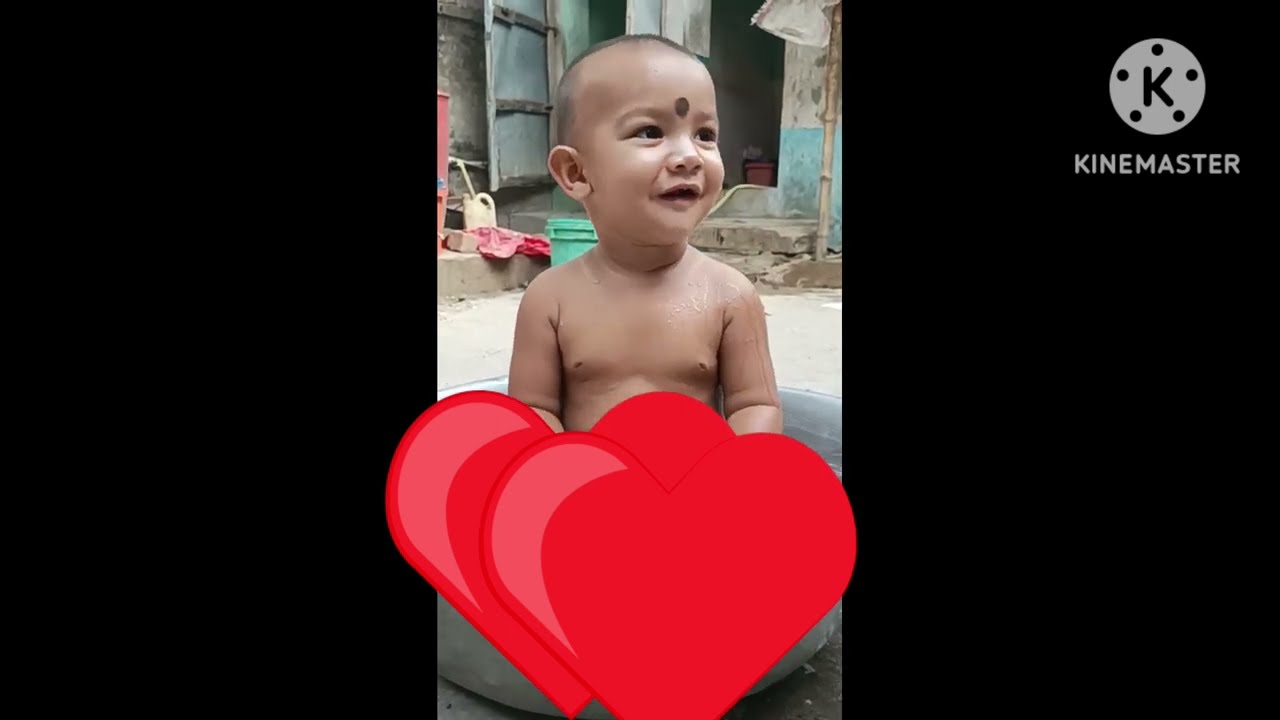The image is a photograph seemingly from Instagram, centered on a young Asian boy who looks to be about two years old. He has no shirt on and from his belly down, the view is obscured by several cartoon hearts, potentially to cover nudity. The boy has light brown skin and a noticeable large brown mole or birthmark in the center of his forehead, between his eyebrows. He is sitting and looking off to the right with an engaged expression, his mouth slightly open in a near-smile. On the upper right corner of the image, we see the watermark "KINDMASTER," with a logo featuring a circle and a "K" inside it. The background suggests a slum or underdeveloped area, with visible details like stones, random pink clothing, a teal bucket, a plastic jug, and an old, leaning door. The photograph appears to have been taken outdoors, possibly during the daytime, with the left and right sides of the frame solid black, likely due to the cropping or framing of the picture.